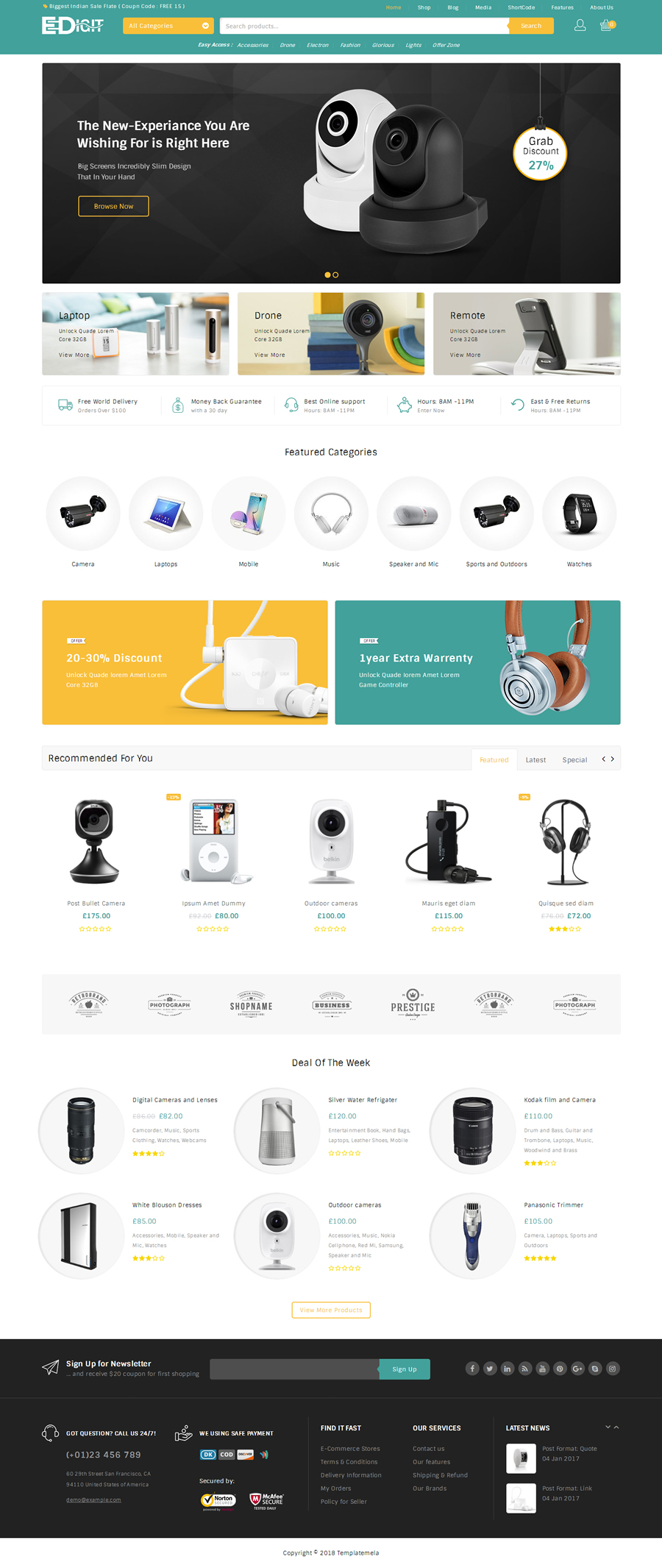This image, taken from a smartphone screen, showcases a vibrant and detailed webpage. Dominating the center of the screen is the text "E Digit, E Digit," with an intriguing visual where the letter "D" morphs into a plug connecting to the letter "E," which features two green areas. 

At the top of the screen is a green rectangular section containing a bright yellow rectangle with the text "All Categories." Moving across this top section, there is a white text field labeled "Search Products," followed by a yellow button labeled "Search." Further along, an icon indicating items in a shopping bag is visible, though the exact digit is difficult to read.

Below this, a black rectangular banner displays the message, "The new experience you are wishing for is right here. Grab discount 27%," styled to resemble a Christmas ornament. Prominently featured just beneath this message is a slogan, "Big screen, incredibly slim design, all in your hand," followed by a "Browse Now" button.

As the viewer's gaze moves down the page, a variety of technology items are displayed, including numerous cameras, indicating a rich selection of tech gadgets available for browsing.